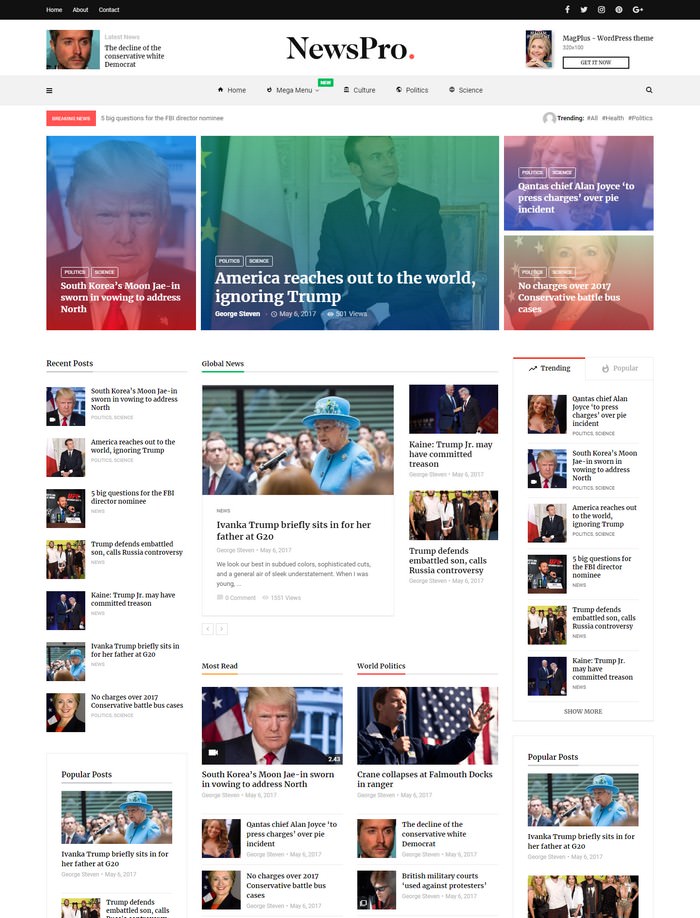The screenshot captures the homepage of a website, presumably "News Pro." The header area stands out with a prominent black strip at the top. On the left side of this strip, navigation options labeled "Home," "About," and "Contact" are displayed. To the right, social media icons for Facebook, Twitter, Instagram, and Google Plus are aligned.

Immediately below the black strip, the background transitions to white, presenting a layout with multiple sections. On the left, there is a photo accompanied by the caption "Latest News: The Decline of the Conservative White Democrat." Next to it, the site’s name "News Pro" is prominently displayed. Toward the right, an advertisement for the "Mag Plus WordPress Theme" urges visitors to "Get It Now."

Below this section lies a horizontal gray line separating the header from the body. Situated to the lower left of this line is a menu icon. Centered within the layout, the word "Home" is followed by a "Mega Menu" drop-down option listing categories such as Culture, Politics, and Science. A search icon is placed on the far right.

The main content area features a bar with four photographs spanning across it. The leftmost photo shows Donald Trump with a caption that reads, "South Korea: Moon Jae-in is sworn in, vowing to address North." The middle image displays a British politician with the text, "America reaches out to the world, ignoring Trump." On the right, there are two stacked photographs. The top image’s caption reads, "Qantas Chief Alan Joyce to press charges over Pi incident." Below it, another image features Hillary Clinton in the background with the caption, "No charges over 2017 conservative battle bus case."